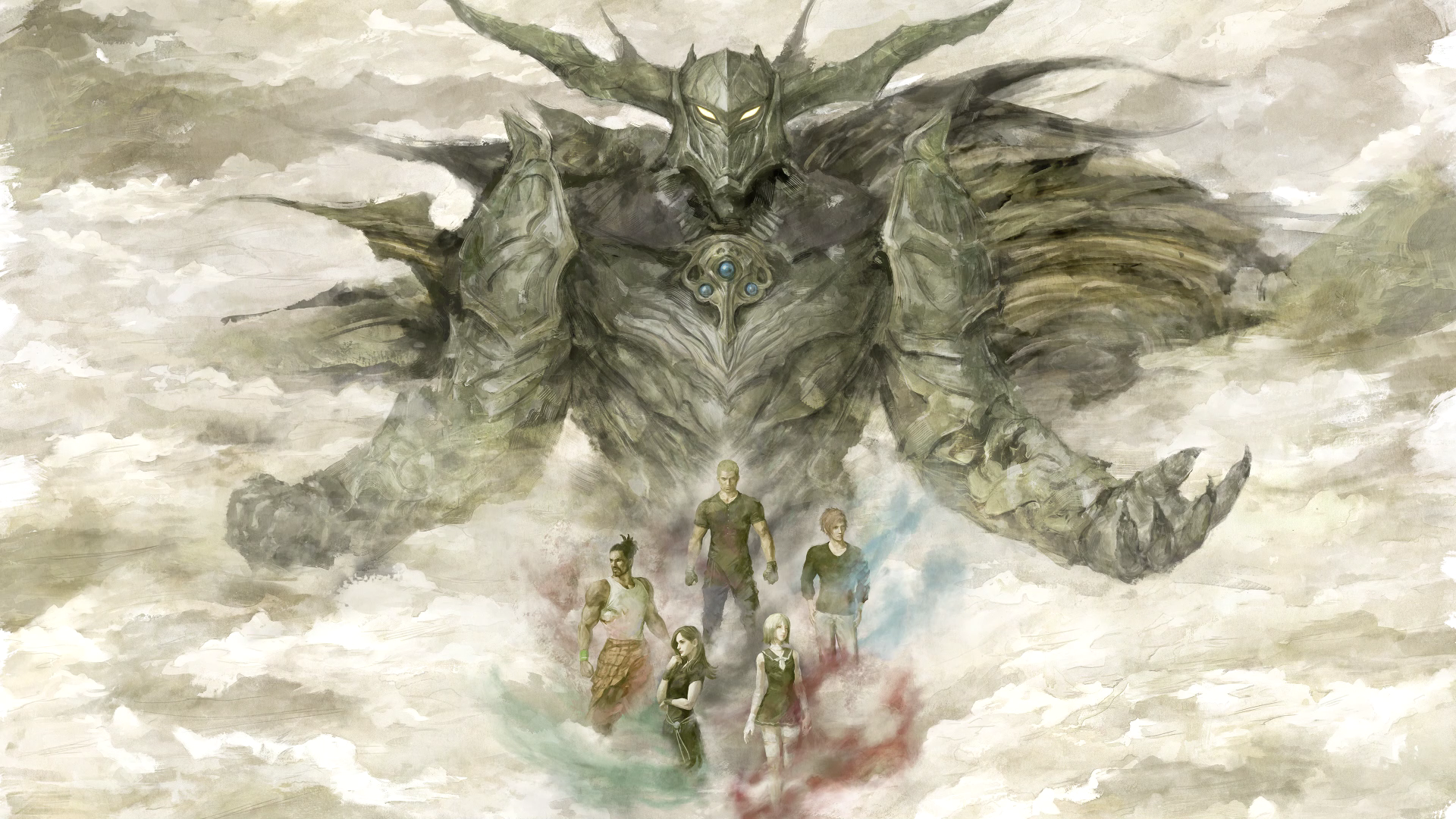This detailed illustration, likely intended for a comic book or teen show, features a monstrous figure rendered in a dramatic, watercolor style. The central figure is colossal and enveloped in an intimidating aura, characterized by dark or olive-green hues. It wears a menacing mask that exhibits glowing, horizontal yellow eyes and large, horn-like extensions. The creature's arms are outstretched—its right hand displaying sharp fingernails in an open palm and its left hand clenched into a fist—creating an imposing and summoning gesture.

The figure’s chest, devoid of legs in the visible frame, is marked with three light blue dots and possibly adorned with metallic plates or scaled armor. Surrounding its chest region, a swirling mist of red, blue, and green clouds add an ethereal and ominous vibe. Below and directly in front of this fearsome being are five humans: two men and three women, one of whom stands with arms folded. Dressed variably, one individual in a tank top showcases pronounced muscles. They are organized in a pentagon formation, amplifying the intricate and dynamic composition of this powerful image.